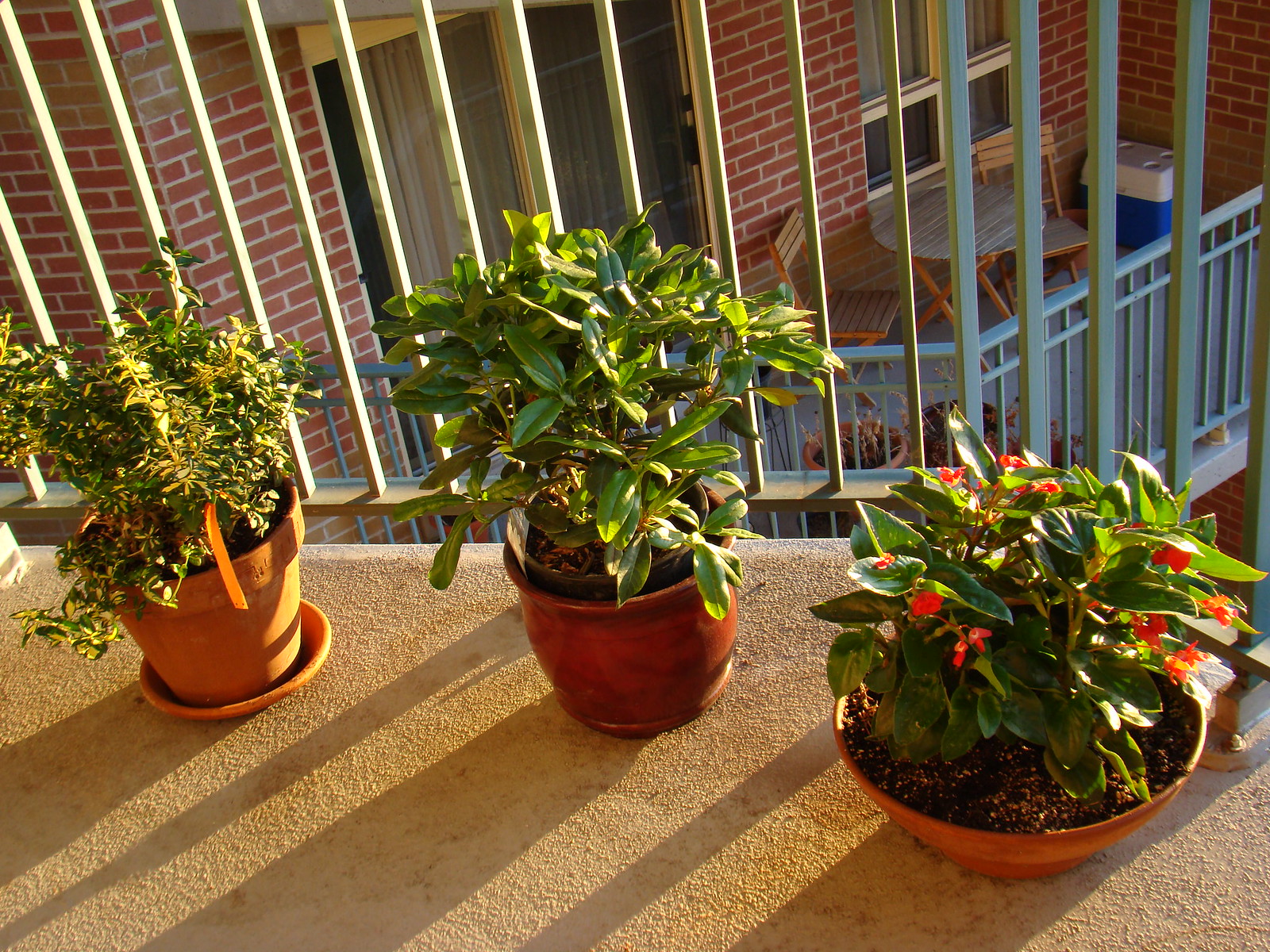On a sunlit apartment balcony with a green metal handrail, three potted plants rest on a textured gray concrete floor, which glows brown due to the sun. The shadows from the terracotta pots add depth to the scene. The left plant sits in a terracotta pot with a matching saucer and features a small bush with relatively thin branches and small oval leaves. The middle plant, a small decorative tree with thicker branches and long, thin leaves, resides in a rounded terracotta pot. The right plant, in a wide terracotta bowl, is a stout green plant adorned with pointy, teardrop-shaped leaves and red flowers. In the background, another balcony below has a small wooden table and two matching chairs, giving a glimpse into the neighboring apartment.